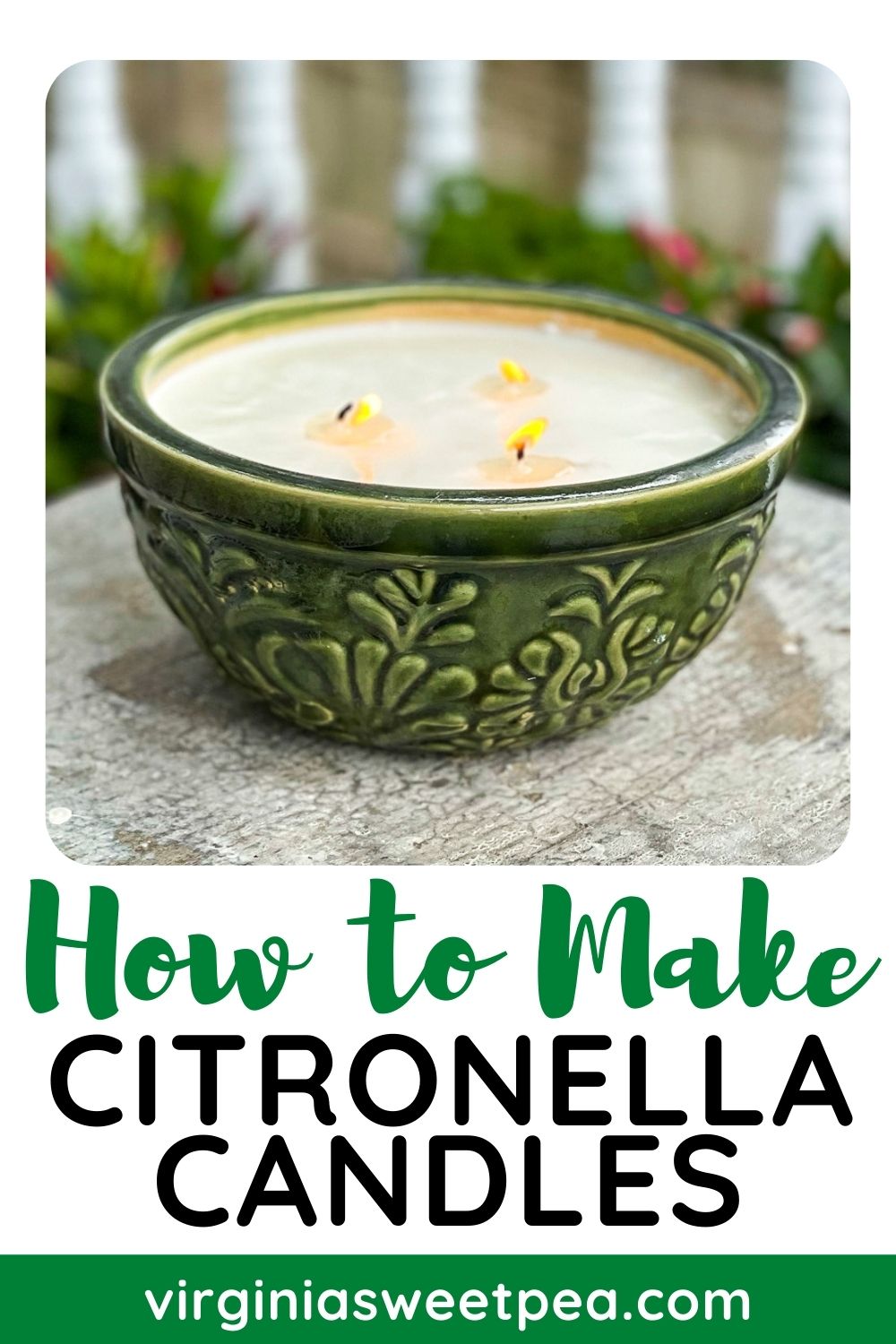The image features a citronella candle housed in an intricately patterned green bowl with three short, lit wicks, placed on a wooden or stone surface outdoors, possibly in a backyard. The background is blurred, revealing bushes, plants, and what appears to be a white house. Above the candle, bold green cursive text reads "how to make," followed by “citronella candles” in black font. At the bottom of the image, inside a green stripe, the text "virginiasweetpea.com" is clearly displayed. The overall layout suggests that this could be the front cover of a magazine.